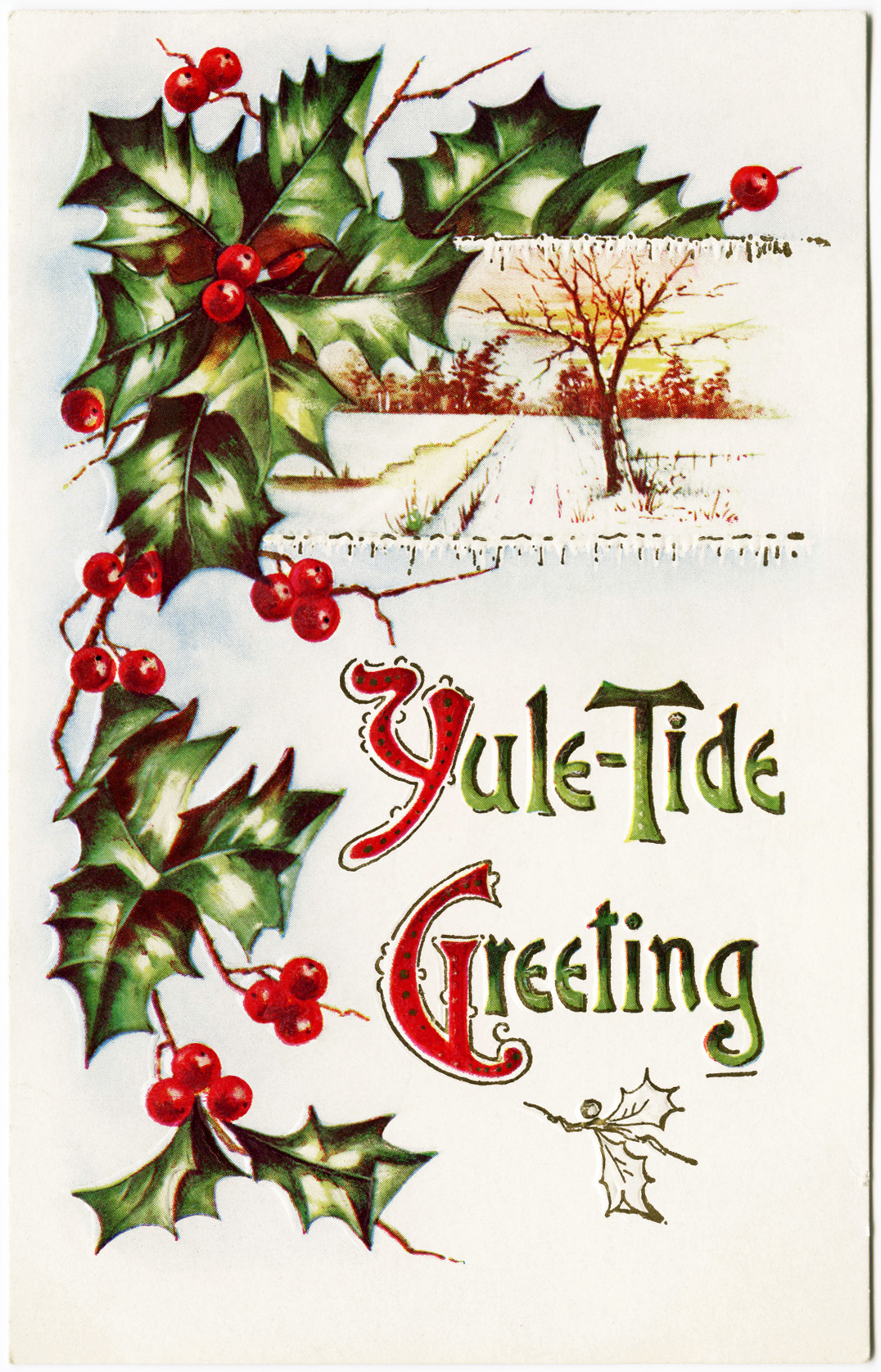This image depicts a Christmas-themed greeting card set against a primarily white background. The card features a charming, old-school design with a mix of illustrations and decorative fonts. The focal point is the text "Yuletide Greeting," displayed prominently in a decorative font. Notably, the first letters "Y" and "G" are in red, while the remaining letters are green, mirroring the colors of the accompanying holly illustrations.

On the left and top borders of the card, there are lush green holly leaves intertwined with vibrant red berries, bringing festive cheer to the design. Above the text, a serene snowy landscape is depicted, featuring a bare tree in the foreground and a forested background with snow-covered pine trees. This countryside scene enhances the nostalgic and minimalistic aesthetic of the card.

Additionally, there is an uncolored mistletoe illustration located beneath the "Yuletide Greeting" text, contrasting with the colored holly. This intricately detailed card harmonizes the traditional Christmas elements of holly, berries, and a snowy winter scene, making it a quintessential holiday greeting.